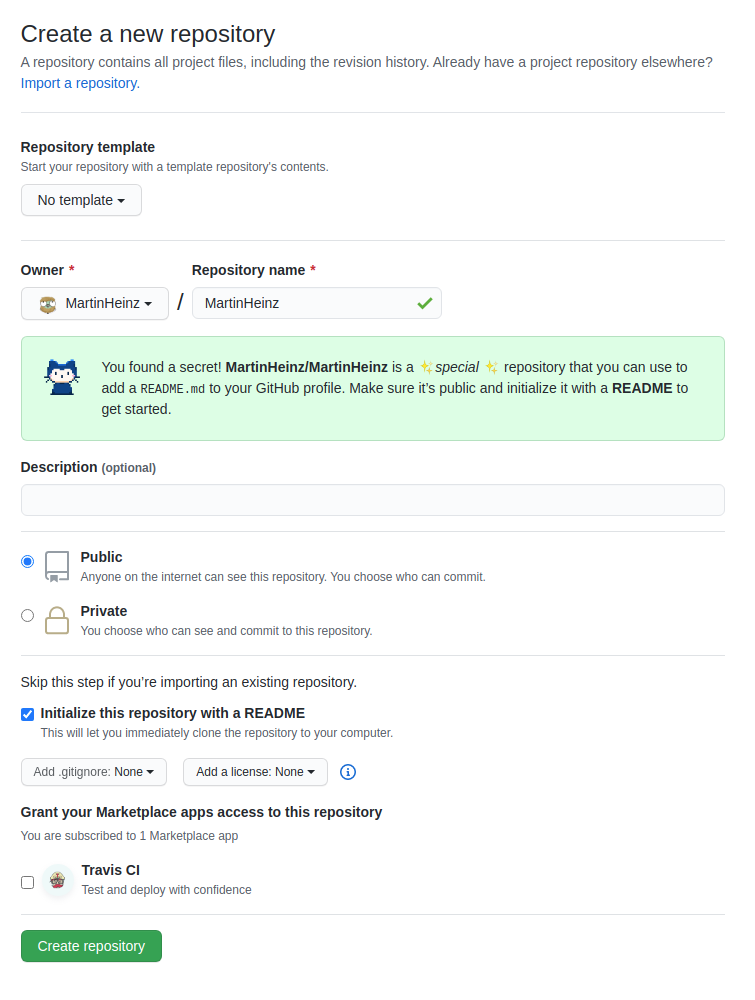This image is a screenshot of a content management software interface, specifically geared towards creating a new GitHub repository.

At the top, there is a header that reads "Create a new repository," followed by a subheader that explains, "A repository contains all project files including the revision history." Below this, there is a note stating, "I already have a project repository elsewhere," which is accompanied by a clickable link to import an existing repository.

The interface is divided into several distinct sections:

1. **Repository Template**: This section features a drop-down menu for selecting a repository template.

2. **Repository Owner and Name**: Here, users can input the name of the repository owner and the name of the repository itself.

3. **Secret Tooltip**: A light blue box with a light blue border contains a tooltip with a small cartoon fox icon, also in blue. The tooltip's text reads: "You found a secret. Martin Hines is a special repository that you can use to add a README.md to your GitHub profile. Make sure it's public and initialize it with a README to get started."

4. **Description Section**: An optional text box allows users to add a description for their repository.

5. **Visibility Options**: Two radio buttons are available:
    - **Public**: Indicates that anyone on the internet can see the repository, but access to commit can be controlled.
    - **Private**: Allows users to choose who can see and commit to the repository.

6. **Initialization Options**: A checkbox to initialize the repository with a README file.

7. **Additional Settings**: Two drop-down menus:
    - **Add .gitignore**: To include a .gitignore file.
    - **Add a License**: To add a license to the repository.

8. **Marketplace Apps Access**: An option to grant marketplace apps access to the repository, with a radio button labeled "Travis CI" for testing and deployment purposes.

Finally, a prominent green button at the bottom labeled "Create repository" enables the user to create the repository with the specified settings.

Overall, the screenshot provides a detailed view of the repository creation process in a content management software interface, capturing all key settings and options.